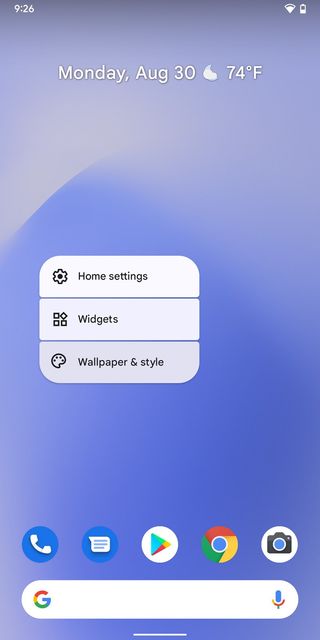The image depicts a detailed screenshot of a mobile device's home screen. The rectangular screenshot is displayed in profile mode, showcasing a standard interface. 

At the top right corner, the status bar contains battery and Wi-Fi icons, while the top left shows the time as 9:26. The background is primarily blue, featuring soft geometric shapes and curves in two distinct shades of blue. Most of the text displayed is either white or black for clarity against the blue backdrop.

Centered towards the top, the date and temperature are displayed in white text, reading: "Monday, August 30, 74 degrees Fahrenheit."

Midway down the screen, there is a distinctive square element with rounded corners, divided into three equal horizontal sections, each with a small gap between them. These sections act as buttons for different functions: "Home settings," "Widgets," and "Wallpaper and style," each accompanied by their respective icons.

At the bottom of the screen, a row of additional buttons is visible, including icons for the phone, Google Camera, and others. There's also a search box placed conveniently for quick access. The overall layout is clean and organized, providing a user-friendly interface.